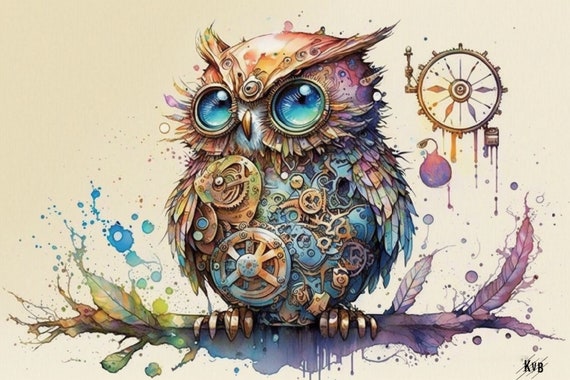The image is a vibrant and detailed painting of an owl with a strong steampunk aesthetic. The owl, adorned with clockwork gears and intricate mechanical parts, has lenses for eyes that shine bright blue. While the inner mechanisms showcase the steampunk theme, the outer layer of its feathers appears relatively normal. The owl sits on a rainbow-colored branch that starts green and brown, transitioning through shades of orange, blue, purple, and red. The branch, and the background elements, have a surreal quality, appearing to dissolve into wax-like droplets and watercolor splotches. To the right of the owl, a cog is depicted melting into nothingness, enhancing the painting’s dreamlike atmosphere. The entire scene is bathed in a mix of purples, greens, and blues, creating a psychedelic aura. The artwork is signed "KVB" in the bottom right corner.